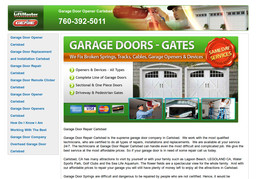### Detailed Caption:

The image is an advertising detail for a website, displayed in a small, landscape (horizontal) format. At the very top of the image, there is a bar that spans the width of the ad. On the far right of this bar, there is a photograph depicting a three-car garage. To the left of this photograph, the background is green with small white text that is illegible, but also includes a clearly visible phone number: **760-392-5011**, notably without parentheses around the area code. On the extreme left side of the top bar, a dark gray or black section houses the company's name and logo, which are unreadable in this image.

Beneath this top bar, the left side features a pale gray column containing 17 lines of blue, presumably clickable, links or menu items.

On the right side of the image, bordered by a thin gray line, there is an advertisement highlighting garage doors and gates. The ad includes a prominent photograph of two white garage doors with arched tops, reminiscent of carriage house gates, although it is unclear whether they swing open or upward. Superimposed on this photograph is a red wax-seal-like graphic, likely indicating "same-day service."

Below the main photograph are three smaller thumbnail images. The first thumbnail on the left shows an installer working on a garage door motor. The second thumbnail appears to display an open garage door, while the third thumbnail's content is indeterminate.

In the lower left corner of the image, various payment method icons are visible, including those for American Express (blue), Visa (blue, white, and yellow horizontal stripes), MasterCard (interlocking red and yellow circles), and another unrecognizable icon.

Below all these elements, several paragraphs of tiny black text on a white background provide additional details, though the specifics of the text are not discernible.